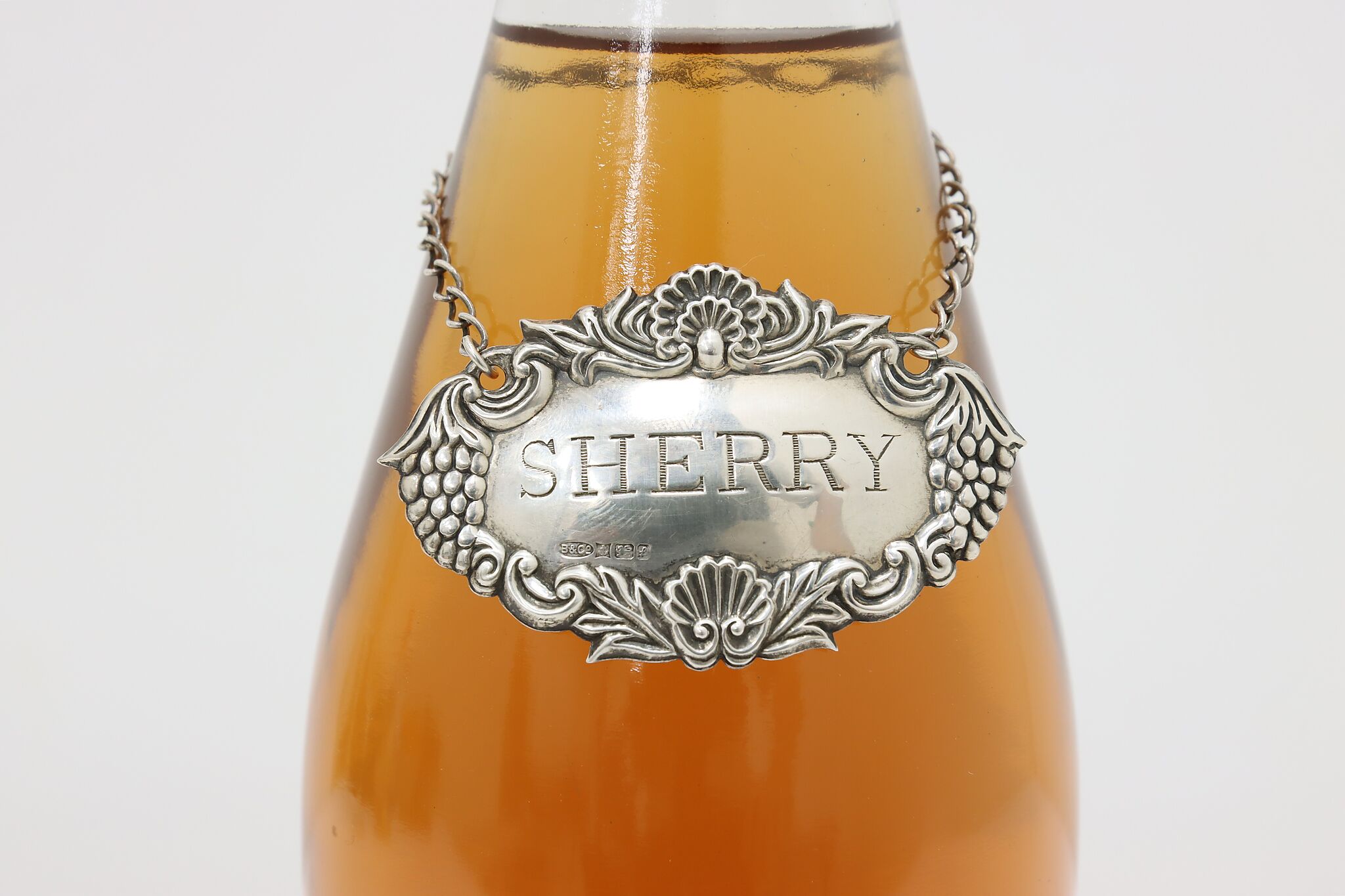This is a detailed color photograph of a sherry bottle set against a light gray background. The bottle contains an amber-colored liquid, reminiscent of apple juice or beer, confirming it is sherry. Around the neck of the clear glass bottle, there is an ornate silver chain-like bracelet. This chain supports an oval-shaped, filigree-patterned medallion, adorned with intricate designs of leaves and grapes. The silver medallion prominently displays the word "SHERRY" etched in capital letters, with some additional smaller text below. The image is closely cropped, emphasizing the bottle's top portion and capturing the elegant details of the medallion and chain. You can distinctly see the liquid level at the very top, as well as glimpses of the chain's backside through the translucent sherry.